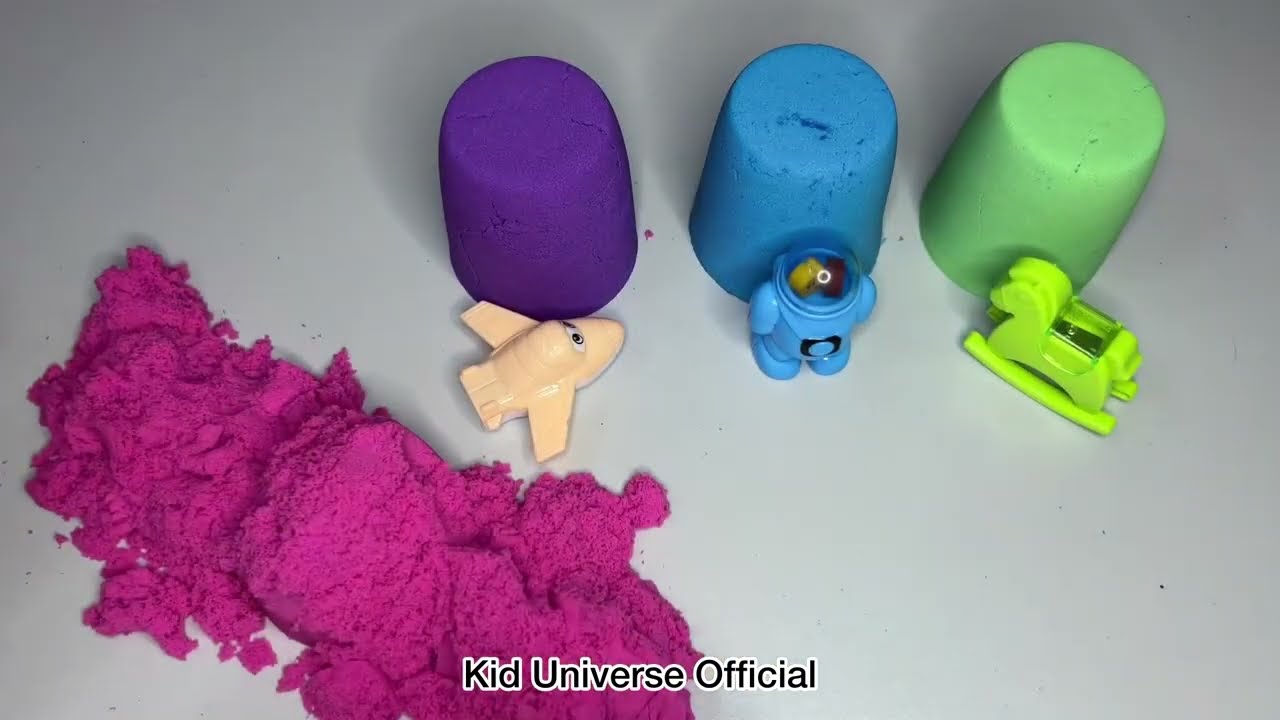This image, likely a still from a YouTube video titled "Kid Universe Official," showcases various playful elements on a white surface. The text "Kid Universe Official" is prominently displayed at the bottom in black, outlined in white. The scene includes four sections of kinetic sand in vibrant colors. The pink kinetic sand is loosely spread across the lower left corner of the image. Three molded sand cylinders—purple, blue, and green—are positioned centrally and towards the upper part of the image. In front of each cylinder, there are corresponding small plastic figurines: a tan airplane is placed before the purple cylinder, a blue astronaut stands before the blue cylinder, and a lime green rocking horse is set in front of the green cylinder. The overall arrangement and vivid colors provide a visually engaging and playful atmosphere, perfect for children's entertainment.